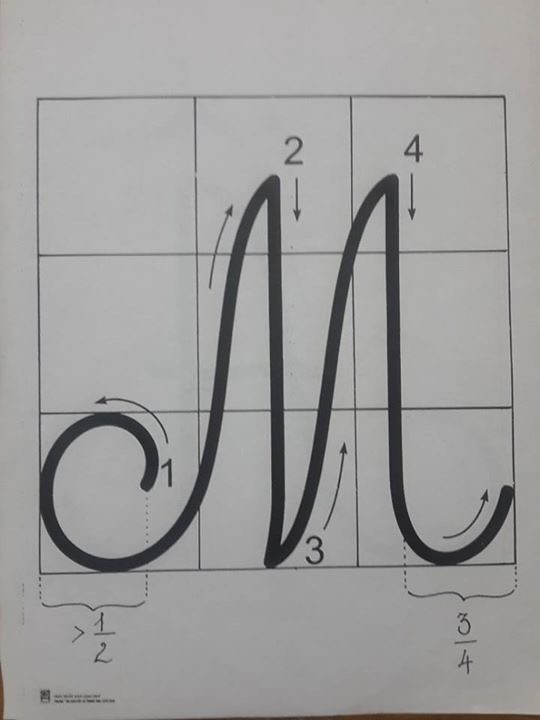This detailed close-up image features a worksheet designed for teaching the cursive letter M, likely intended for elementary school children. The worksheet is divided into a 3x3 grid, offering a structured and geometrical approach to mastering the stylish and almost cursive form of the letter. The M is broken down into four distinct steps, each marked with numbers and arrows to guide the learner's pen or pencil movement. The first step shows a round loop that ascends to the top of the first arch, followed by instructions that guide the flow down to the bottom half of the grid, and then back up and down again, creating elegant curves and loops. Each segment of the grid helps maintain consistent proportions, with annotations like "1/2" and "3/4" suggesting the recommended widths. The sheet is white with meticulous step-by-step diagrams, making it an effective educational tool. There is also some text at the bottom left corner, though it is not clearly visible in the image.